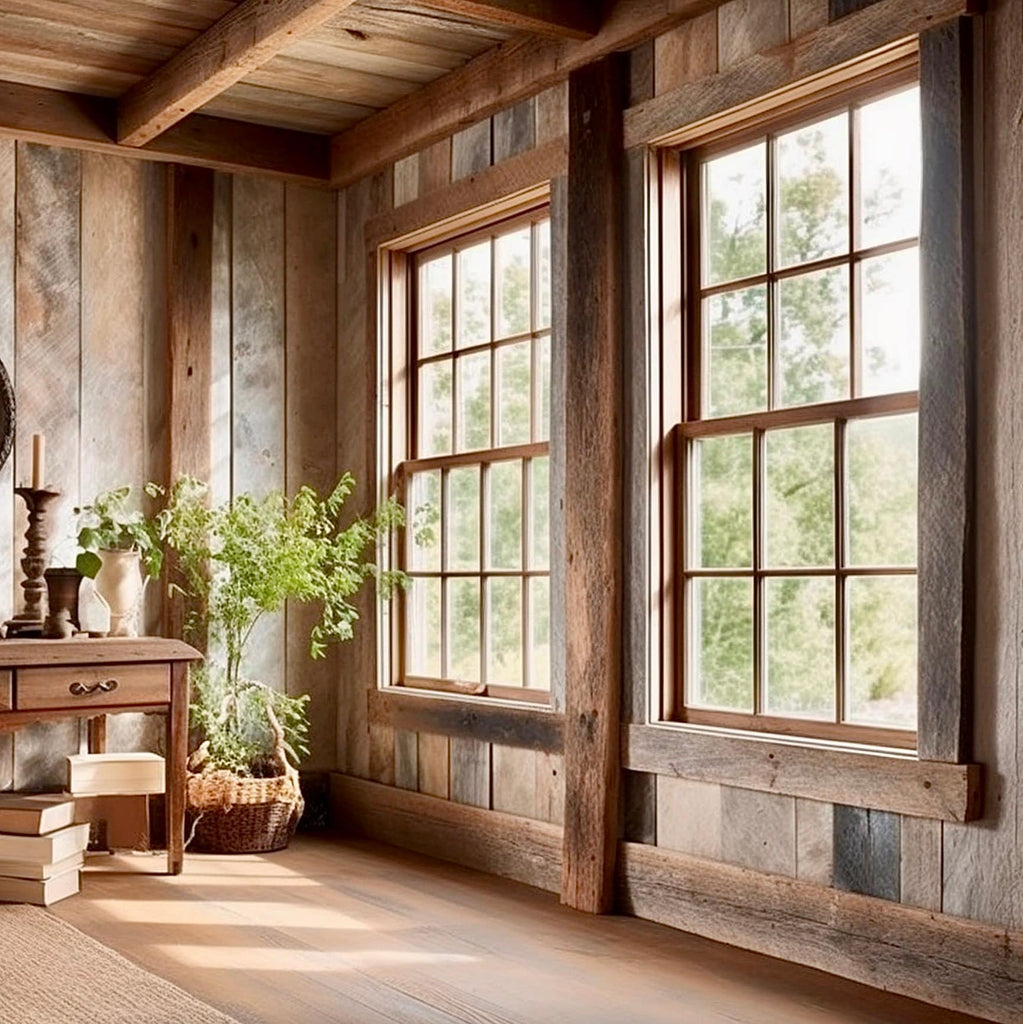The photograph depicts a staged, rustic interior of a cozy, woodsy cabin. The room features a wooden ceiling with planks and slim wooden beams, complemented by light beige hardwood flooring and a tan woven rug. The walls are adorned with large vertical wooden planks in varying shades of brown, exuding a warm, natural atmosphere. Two large windows are positioned on the right wall, each divided into twelve panes, with the left window uniquely featuring sixteen panes. These windows are separated by a dark brown vertical wooden beam and allow natural light to filter in, revealing a view of lush green trees outside.

In the corner of the room, a wicker basket holds a green tree, approximately four feet tall. Adjacent to the tree, a small wooden table displays a brown candlestick with a tan candle, and several books are neatly stacked beneath it. The overall setting suggests a thoughtfully designed space, evoking a sense of tranquility and connection to nature, characteristic of a serene woodland cabin.